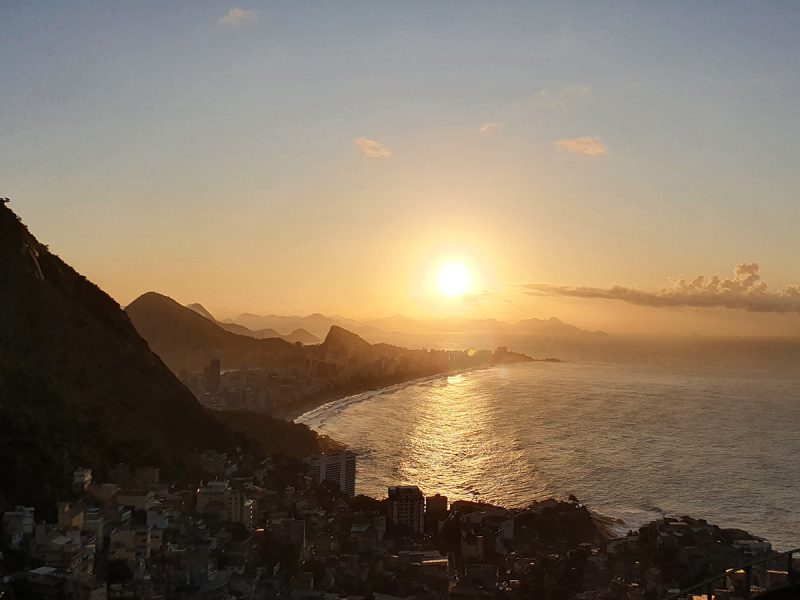This aerial photograph captures a coastal city nestled at the base of a mountain basin. To the right of the city, a vast ocean stretches into the distance, the far shore unseen. The skyline features a cluster of tall, varied skyscrapers mostly shaded in oranges and whites, their hues dimmed by the late afternoon shadows. The sun, centrally located in the image, is setting, casting a golden-orange gradient across the sky and forming a line of reflective light on the bay. A bright blue hue pervades the sky, punctuated by small clouds and a large puffy gray cloud in the bottom right. Behind the city, mountainous ridges extend into distant obscurity, merging with the skyline and creating a scenic backdrop that accentuates the rugged terrain and urban density. The buildings range from dark silhouetted structures to dense clusters of beige and white housings, magnifying the city's architectural diversity.